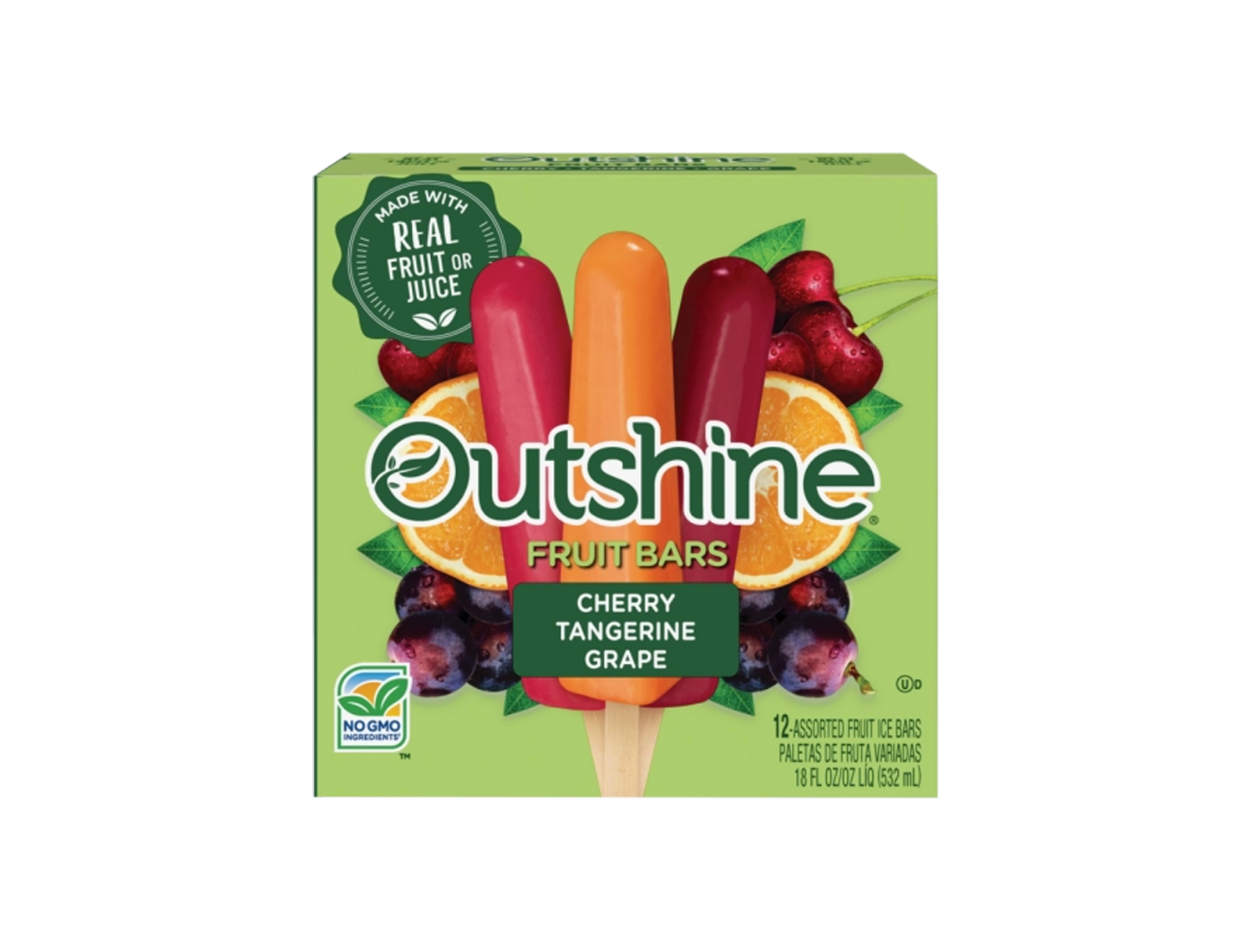The image depicts a light green cardboard box of Outshine fruit bars, prominently showcasing vibrant colors and a mouth-watering assortment of fruit popsicles. The box, viewed from the side, features a bold green stamp declaring "Made with real fruit or juice" alongside a logo indicating "No GMOs." The packaging highlights a picturesque background of cherries, grapes, blueberries, raspberries, and oranges. In front of this fruit array are three distinct popsicles: a lighter red one representing cherry, an orange one, and a darker red one signifying grape. The front of the box clearly labels these flavors as cherry, tangerine, and grape, boasting a total of 12 assorted fruit ice bars amounting to 18 fluid ounces. The popsicles are single-sized with rounded tips, visually appealing against the lively, fruit-themed backdrop that emphasizes their natural and wholesome ingredients.